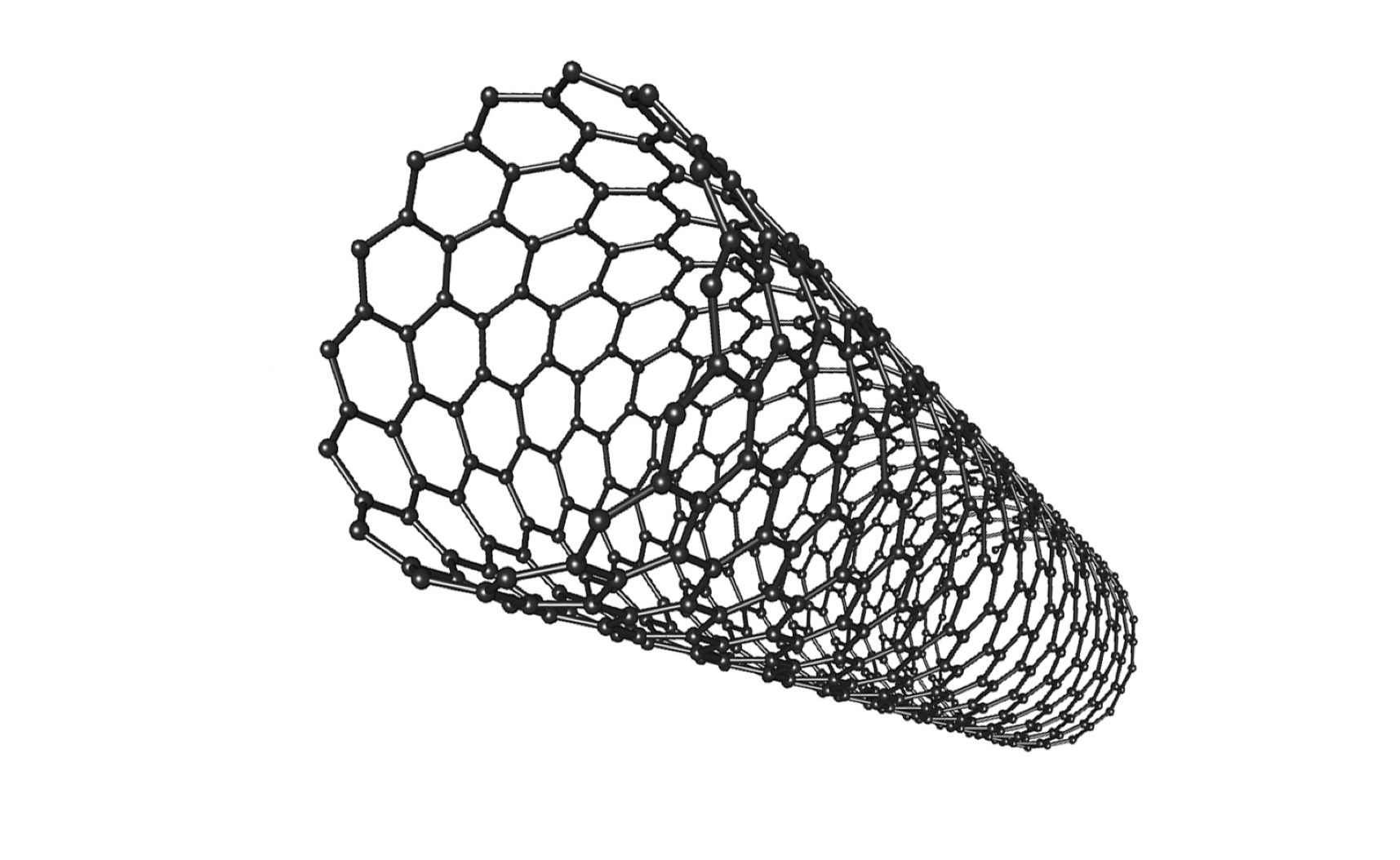The image depicts an intricate, hand-drawn illustration of a large, cylindrical molecular structure against a pure white background. The structure resembles a tightly rolled-up metal mesh or chain-link fence made of repeating hexagonal patterns, similar to those found in chemistry textbooks. Each hexagon is formed by small black dots representing atoms connected by lines, suggesting chemical bonds. The mesh appears to stretch from the top left of the image, where it is closest and most pronounced, to the bottom right, where it gradually diminishes in size, creating a sense of depth. The detailed depiction of interconnected hexagonal units conveys the geometric complexity and precision of the structure.